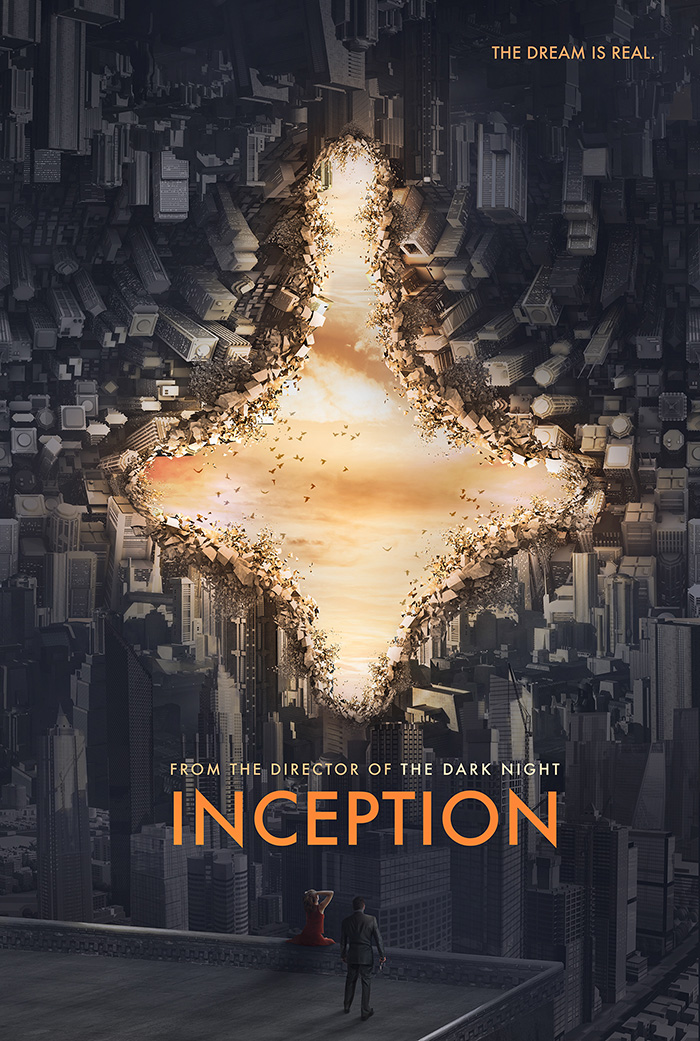This movie poster features the word "Inception" in large, orange, sans-serif font at the bottom, with the subtitle "From the director of The Dark Knight" above it. The slogan "The Dream is Real" is positioned in the top right corner, also in orange sans-serif font. The image portrays a surreal cityscape with gray skyscrapers that appear to be crumbling away, exposing areas with a brownish outline where pieces have fallen off. The entire city is depicted as folding in on itself, creating a dream-like, twisted view, with buildings appearing upside down in all directions. Towards the bottom of the poster, a young woman is sitting on the edge of a building's rooftop while a young man stands nearby, both gazing at the distorted cityscape. The sky is torn apart in a glowing, yellowish, cross-shaped pattern, illuminating the otherwise dark city. Birds can be seen flying within the open sky section. This poster, likely a fan creation, captures the essence of the film's surreal and mind-bending themes.